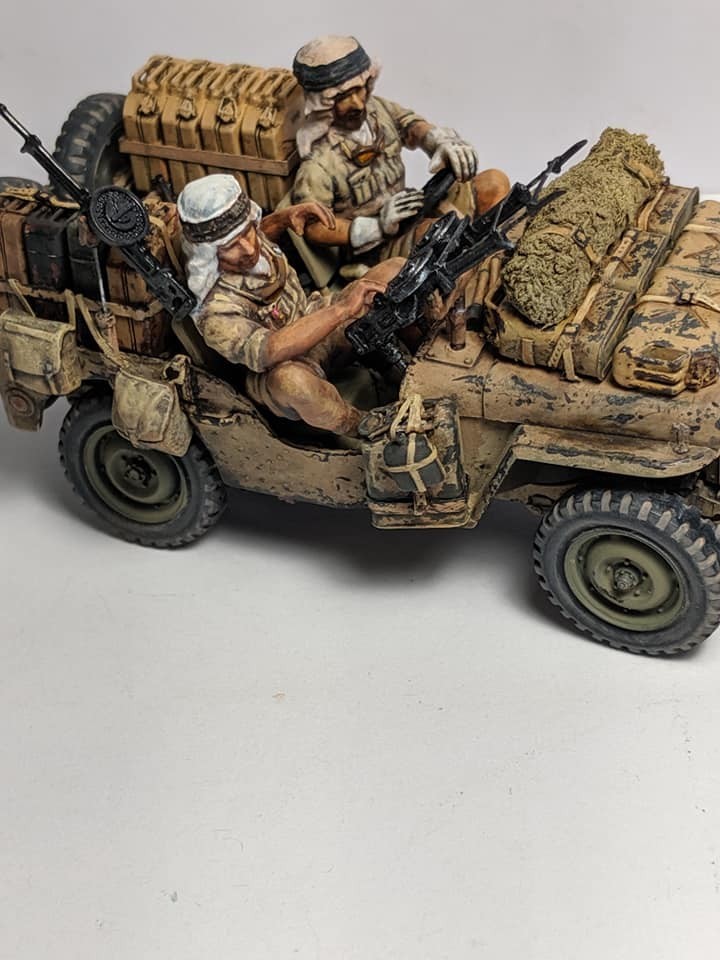The image features a meticulously detailed, scale model of an early 1940s military jeep, captured on a white surface, suggesting it's sitting on a table indoors. The jeep, painted in a blend of beige, tan, and army green, is occupied by two miniature figures dressed in military uniforms. Both figures are wearing green shorts and rolled-up sleeves, indicative of military garb, complemented by green army gear and Middle Eastern-style headdresses that are long in the back with bands around the forehead. Each figure sports a beard and holds a vintage-looking machine gun with distinctive round metal components.

The driver is positioned on the right side, gripping the steering wheel, while the passenger cradles his weapon in his lap. Behind the figures, mounted on the jeep, is a large black gun pointing upwards, accompanied by various cases of equipment, four gas cans, and a spare tire secured at the back. The well-crafted model radiates an aura of authenticity, with shadows visible underneath, enhancing its lifelike appearance against the plain white background.